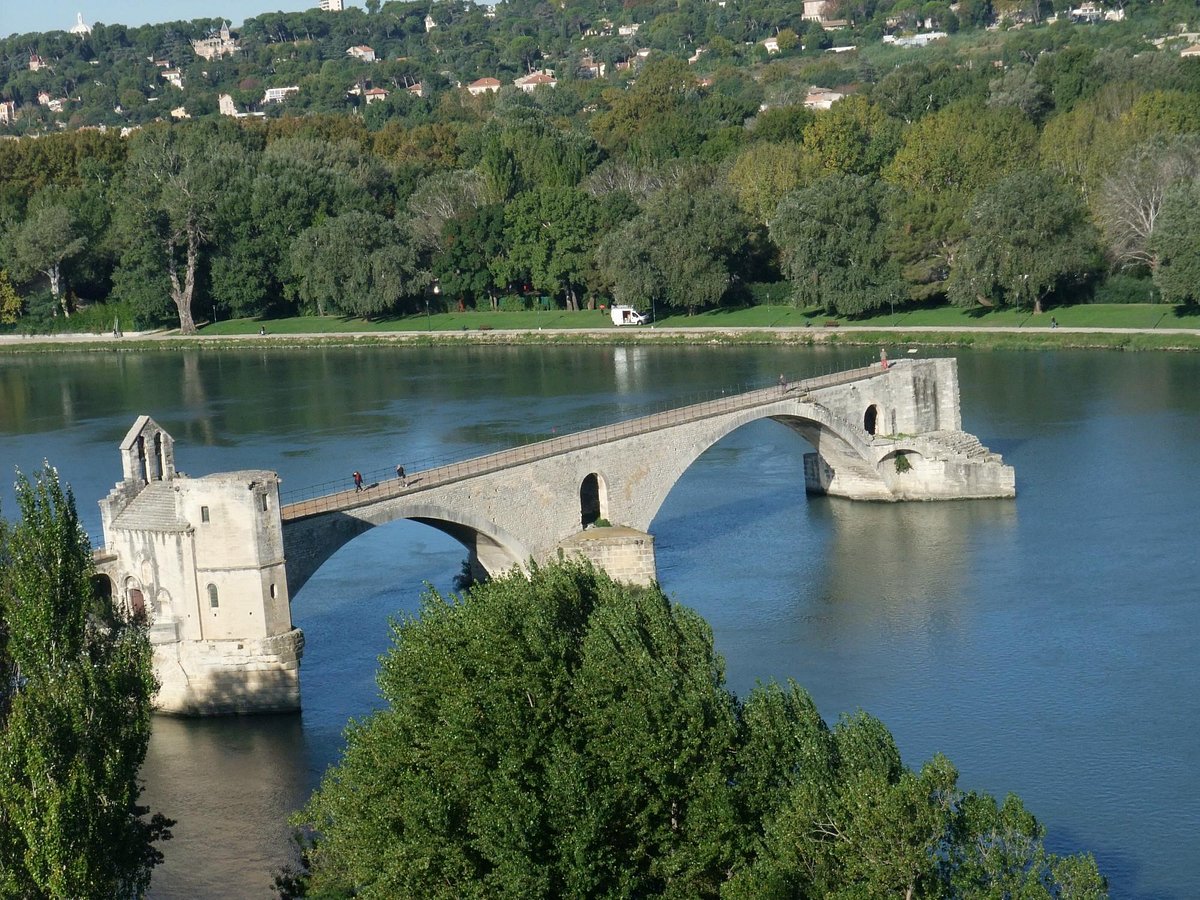The photograph captures an ancient stone bridge with intricate stonework, extending halfway out into a serene river. At the far end of the bridge, an observatory tower stands prominently, with steps leading down, possibly for boarding boats or other water vessels. On the bridge, two people can be seen walking, while another person is at the observatory. The bridge, constructed from sturdy stone, blends its historical charm with the surrounding landscape. The riverbanks in the background feature a lush strip of forest lined with rows of trees, and in the distance, there are visible houses and a quaint village. A white van can be spotted driving along a road on the far side of the river. In the foreground, green bushes frame the scene under the bright, shining sun.